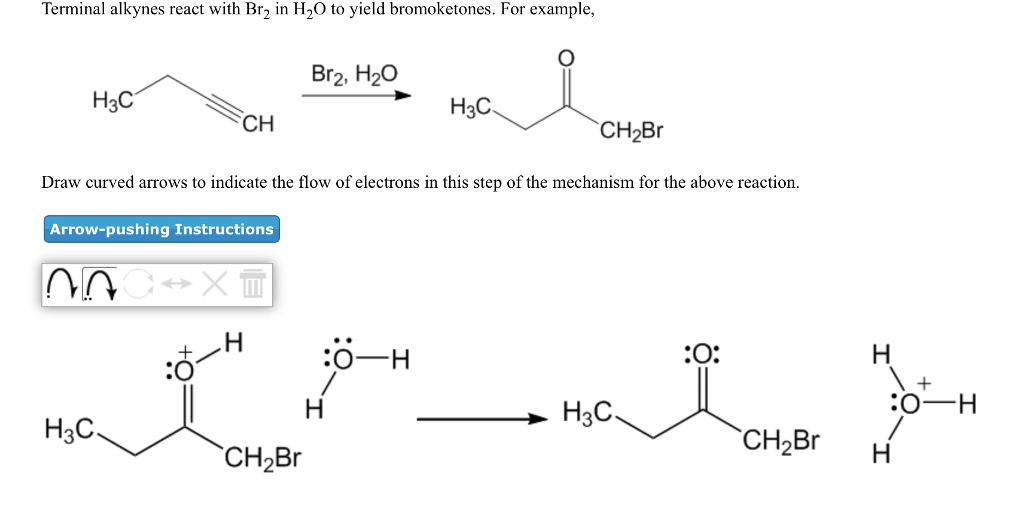The image is a detailed chemistry chart illustrating the reaction of terminal alkynes with Br2 and H2O to yield bromo ketones. At the top, the text reads, "terminal alkynes react with Br2 and H2O to yield bromo ketones." Below this, chemical structures are shown: H3C linked by lines to CH, with a black arrow pointing right to indicate the reaction facilitated by Br2 and H2O. The products are depicted as H3C connected to CH2Br, with double lines indicating an oxygen atom between them. A subsequent section provides instructions: "draw curved arrows to indicate the flow of electrons in this step of the mechanism for the above reaction," accompanied by a blue box labeled "arrow push and instructions." The bottom contains additional chemical formulations and elements, enhancing the depiction of the reaction mechanism.